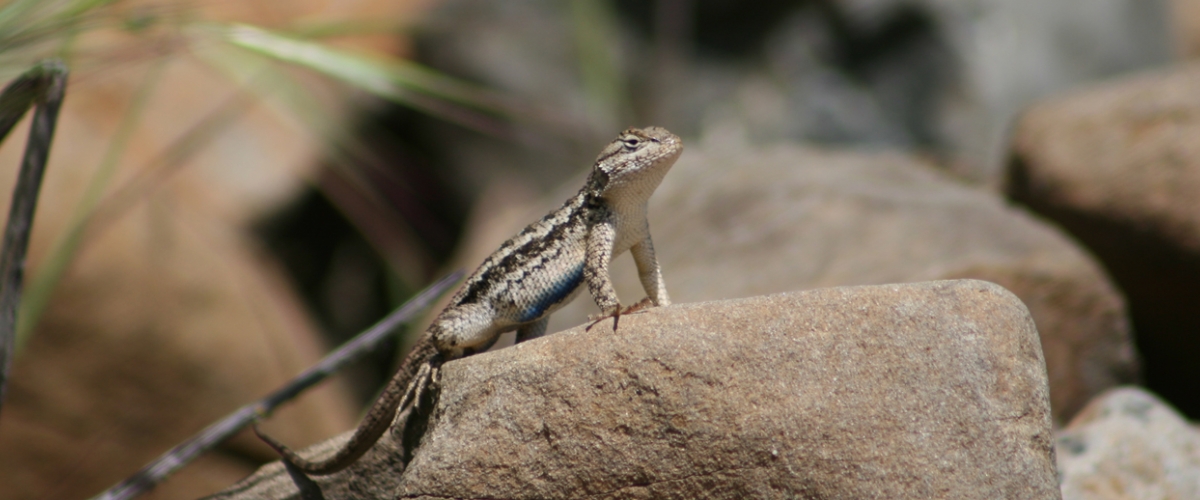This close-up nature photograph captures a beige lizard with a dark brown pattern perched prominently on a pebbled rock in the foreground. The lizard is positioned in a push-up stance, with its two front legs at the edge of the rock and its back legs secured on the surface. It features a beige underbelly with hints of blue, and its back is adorned with dark brown stripes. The lizard's long, mostly brown tail extends outward toward the left, while its head faces up and to the right with a contemplative expression. The rock, variegated in beige, brown, and gray tones, dominates the image along with the lizard. The background is blurred, consisting of indistinct green foliage and additional rocks, lending a shallow depth of field that keeps the focus on the lizard and its immediate perch.